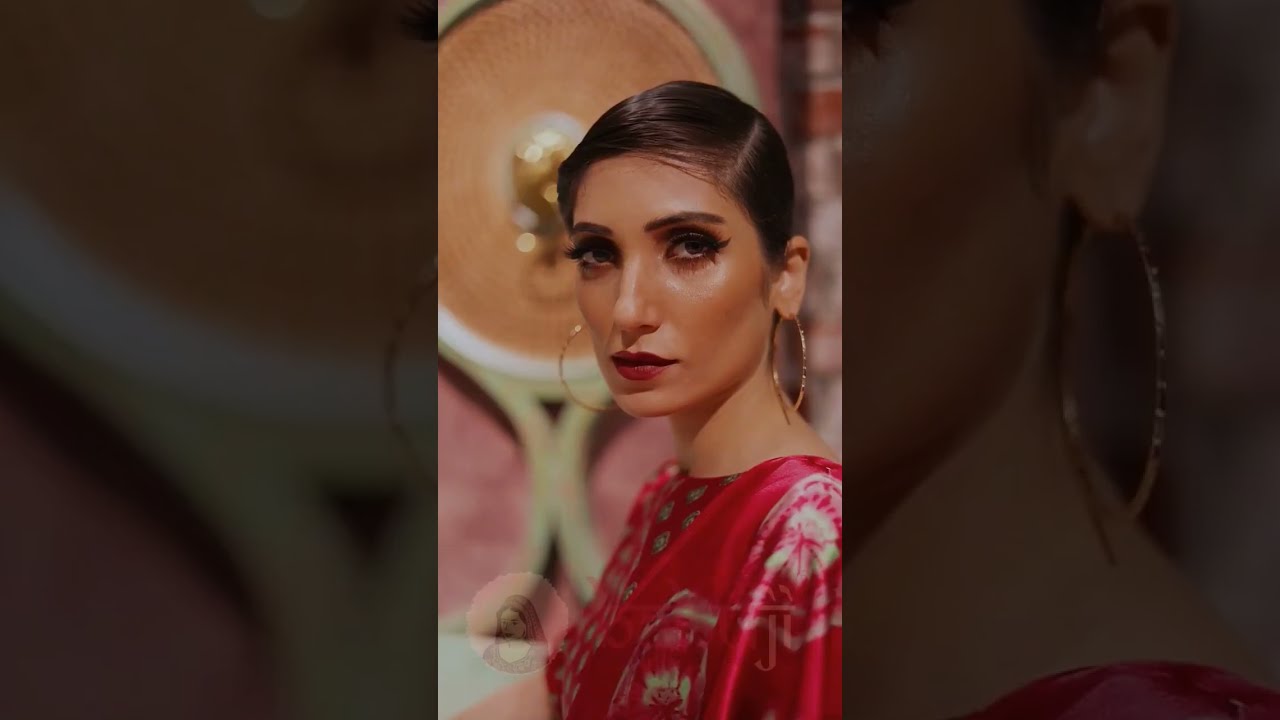A captivating photograph of a woman, likely of East Indian descent, wearing a vibrant red top adorned with green and white floral patterns. Her outfit has a silky, shiny appearance. She accessorizes with large, thin gold hoop earrings, and her makeup is meticulously applied with prominent eyeliner and bold red lipstick, highlighting her enigmatic expression. Her short brown hair is styled neatly, complementing her overall look. She stands in front of an ornate wall fixture resembling a gong, which adds an intriguing backdrop to the photo. The room's background is blurred, drawing attention to her poised demeanor. In the bottom left corner of the image, there is a circular icon of a historical woman dressed in a traditional robe, adding a layer of mystery to the scene. The photograph, presumably taken with a cell phone, features dark sections on either side, further emphasizing the central figure and her striking appearance.